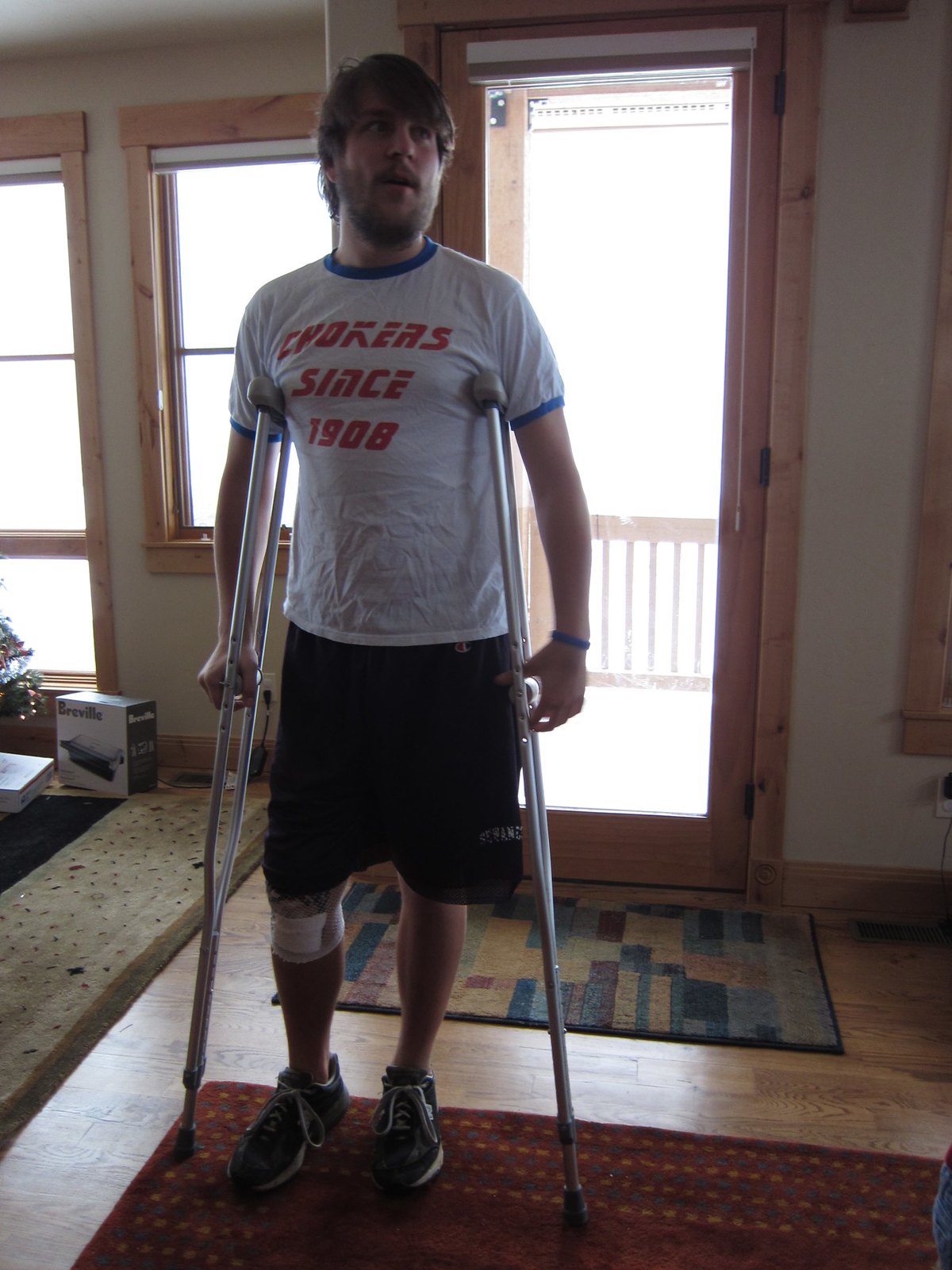In this indoor photograph, a man with a short trimmed beard and messy brown hair stands using silver crutches, indicating he has a leg injury. His left leg is wrapped in a bandage just below the knee and covered with plastic. He is dressed in a white ringer T-shirt with blue trim around the collar and sleeves, which is wrinkled and partially obscures the red text that appears to say "Chokers since 1908." Additionally, he wears black gym shorts, dark sneakers, and a blue wristband on his left wrist. The setting shows a mix of carpet and hardwood flooring, a window, a doormat, and a box that resembles an appliance packaging, adding context to the indoor environment.